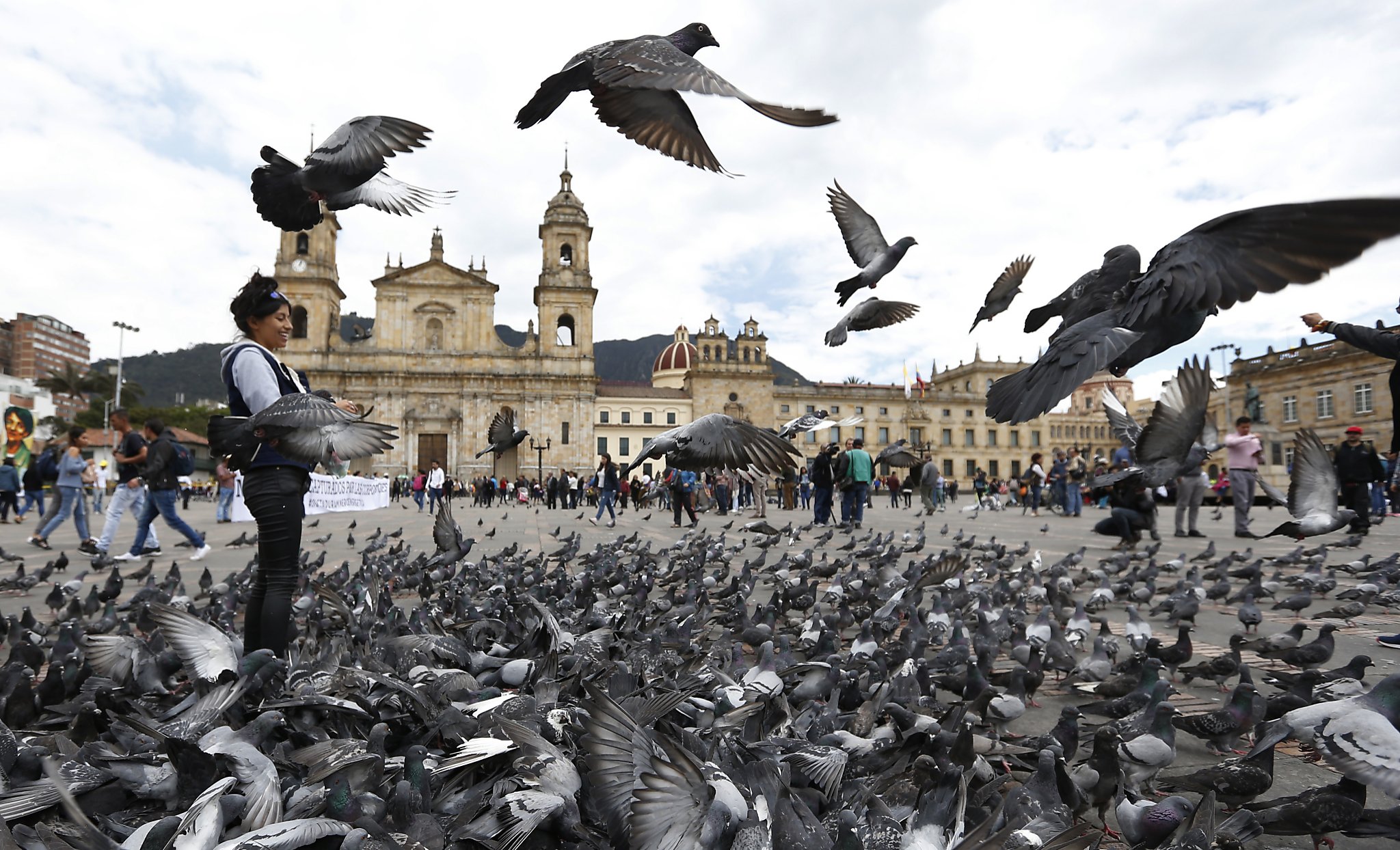In this daytime, color photograph, the setting is the bustling Plaza de Bolívar in Bogotá. The image, in landscape orientation, captures a lively scene where hundreds of pigeons are flocking on the ground and in flight around the open square. People meander in various directions, seemingly unaware of the photograph being taken. Central to the image is a man on the left, dressed in black pants, a black vest, and a white shirt. He smiles while feeding the pigeons, which are densely gathered around him, as well as flying overhead. Dominating the background is a palatial building with a dramatic beige stucco finish, featuring two spire towers flanking the entrance and a gabled pediment above. The building's facade includes three rows of numerous windows and an elongated section on the right capped with a domed roof. The style of the photograph is representational realism, capturing the intricate details and the dynamic energy of the square.